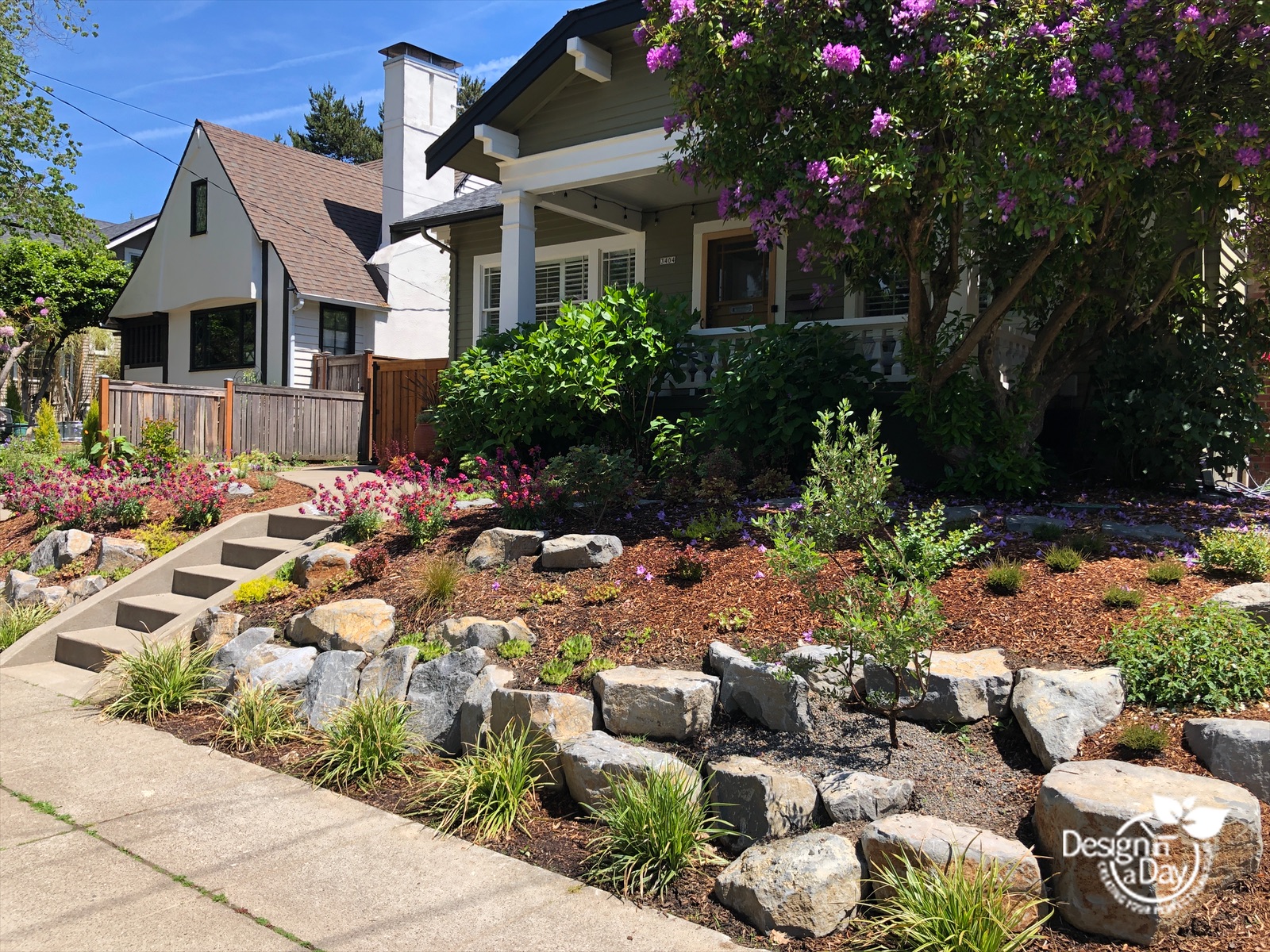This colored photograph captures a suburban or small-town street scene featuring two adjacent houses. The focal point is a charming gray bungalow with white trim and a unique, xeriscaped front yard situated on a sloping grade. The yard, devoid of grass, is beautifully adorned with large, chunky rocks—some reaching up to a foot high and wide—and interspersed with various low-water plants, including small tree-like shrubs, green bushes, and a blooming crepe myrtle with purple flowers. A prominent lilac bush adds to the vibrant landscape, which also includes a set of six stairs descending from the house down to the sidewalk. To the left of the gray house is another residence painted white with a light red roof, accompanied by its own lush garden. Notably, the image bears a watermark in the lower right corner with the logo "Design in a Day."